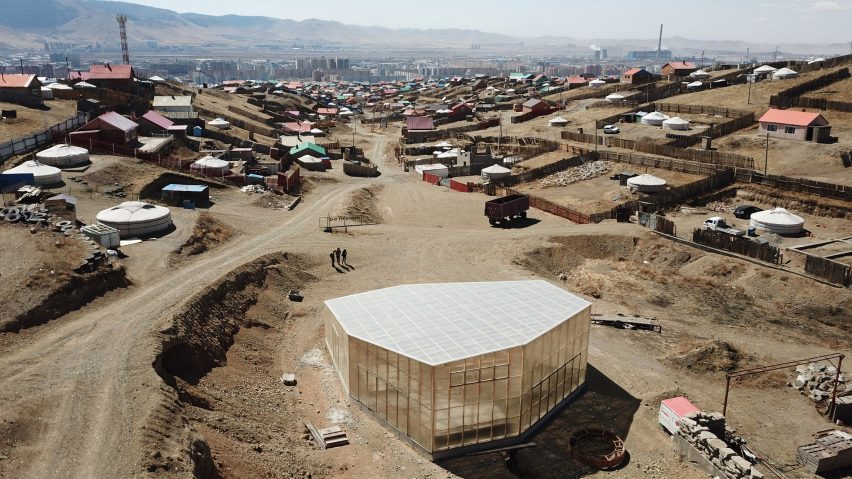This aerial photograph captures a construction site in a barren desert region, characterized by its expansive dirt landscape void of any vegetation. The view shows a central large, unfinished building that stands out with its irregular polygonal shape, wrapped in clear material with rectangular panes, hinting at a greenhouse. This building is surrounded by smaller temporary structures and sectioned off areas, possibly property plots. A dirt road branches from the bottom left corner, diagonally cutting through the middle of the image, and splits into various unfinished paths. Scattered around are trucks and occasional people, highlighting the ongoing development. Further back, the setting transitions into a densely populated town and then into a cityscape, with red-roofed and circular buildings, eventually blending into a slightly foggy, brown mountainous backdrop. The overall scene has an industrial feel, with a sense of organized chaos amidst the dusty, dirt-filled landscape.